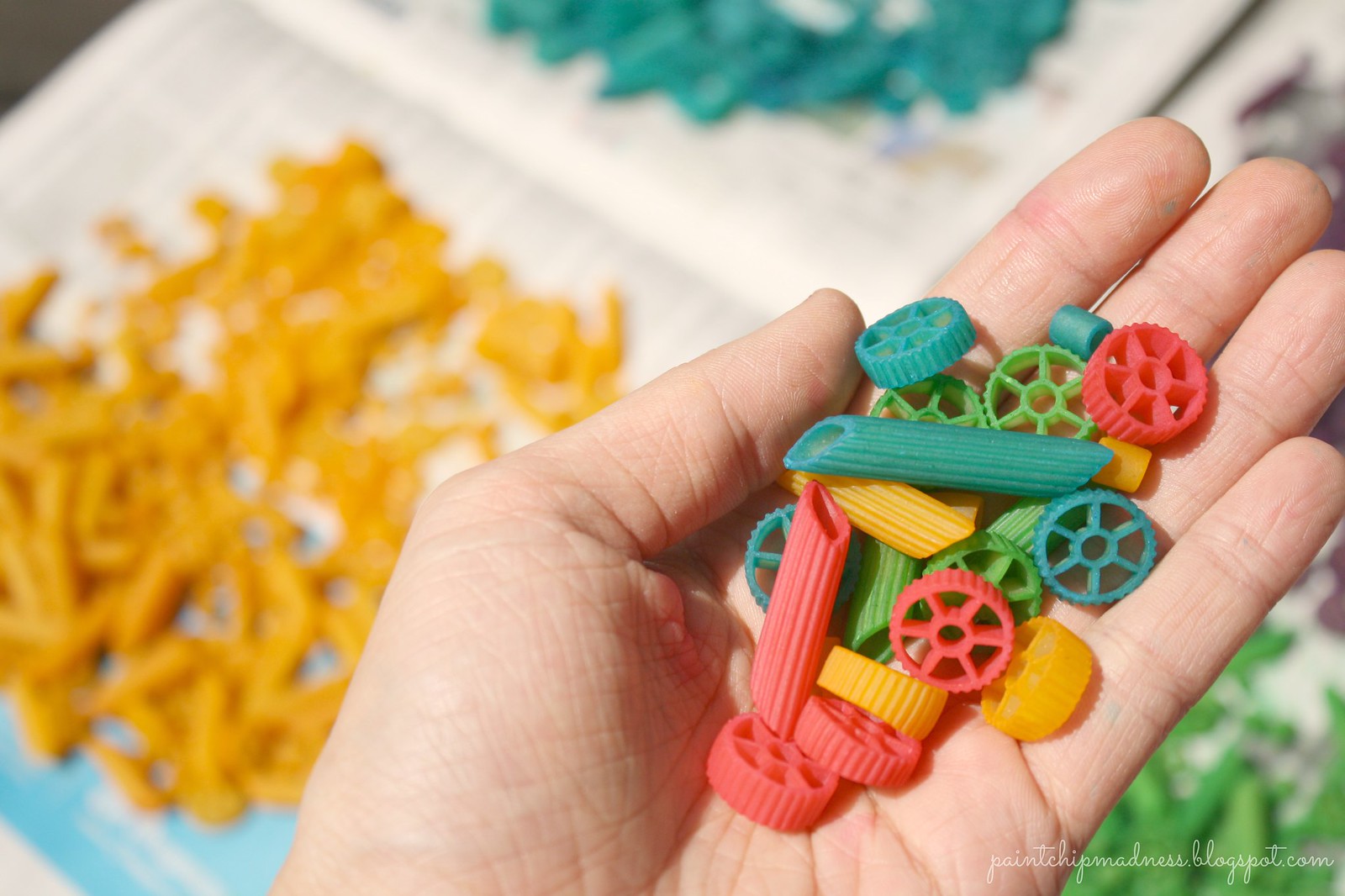In this detailed image, a feminine, white hand is prominently holding a bundle of uncooked, multicolored pasta, featuring penne and wheel shapes. The colors of the pasta held include blue, green, red, and yellow, with some unique bluish-pink hues. In the background, slightly blurred, there are white dishes with assortments of the same colored pasta—yellow to the left, blue above, and green below to the right. Each plate showcases a variety of pasta shapes, emphasizing the vibrant and playful array seen in the hand. Additionally, there are small circular noodles in blue and yellow among the collection. The overall composition draws attention to the diverse shapes and striking colors of the pasta held in the hand, while subtly indicating more varieties on the blurred dishes in the background.